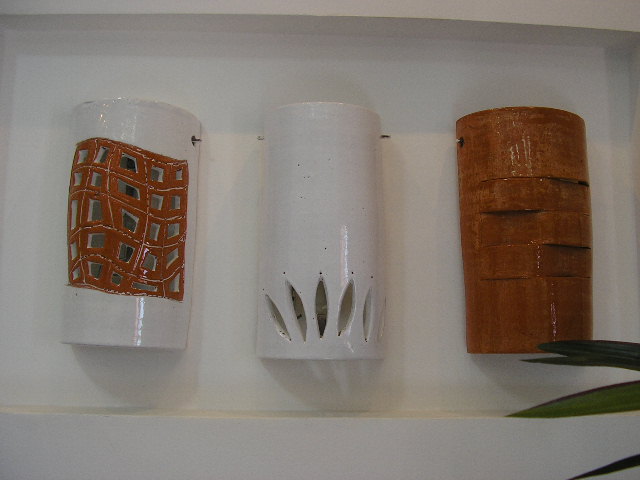This photograph captures three distinctive wall sconces, crafted from glazed porcelain, arranged in a row on a white wall. Spaced about three fingers apart, these sconces are cylindrical or half-cylindrical in shape, designed to provide an ambient uplight or downlight effect through various artistic cutouts.

The leftmost sconce features an elegant combination of white and brown. It has a brown center bordered by a white frame, and is adorned with irregular rectangular cutouts, arranged in a wavy grid pattern allowing light to shine through. 

The middle sconce is completely glazed in glossy white and showcases petal-shaped slits near its bottom, reminiscent of pea pods, offering a unique way for light to diffuse.

The rightmost sconce is entirely coated in a rich brown glaze, structured with horizontal slits that give a woven appearance similar to a pie crust, creating a checkerboard effect for light to escape. Additionally, three leaves are depicted at the bottom right of the image, suggesting a touch of nature added to the design.